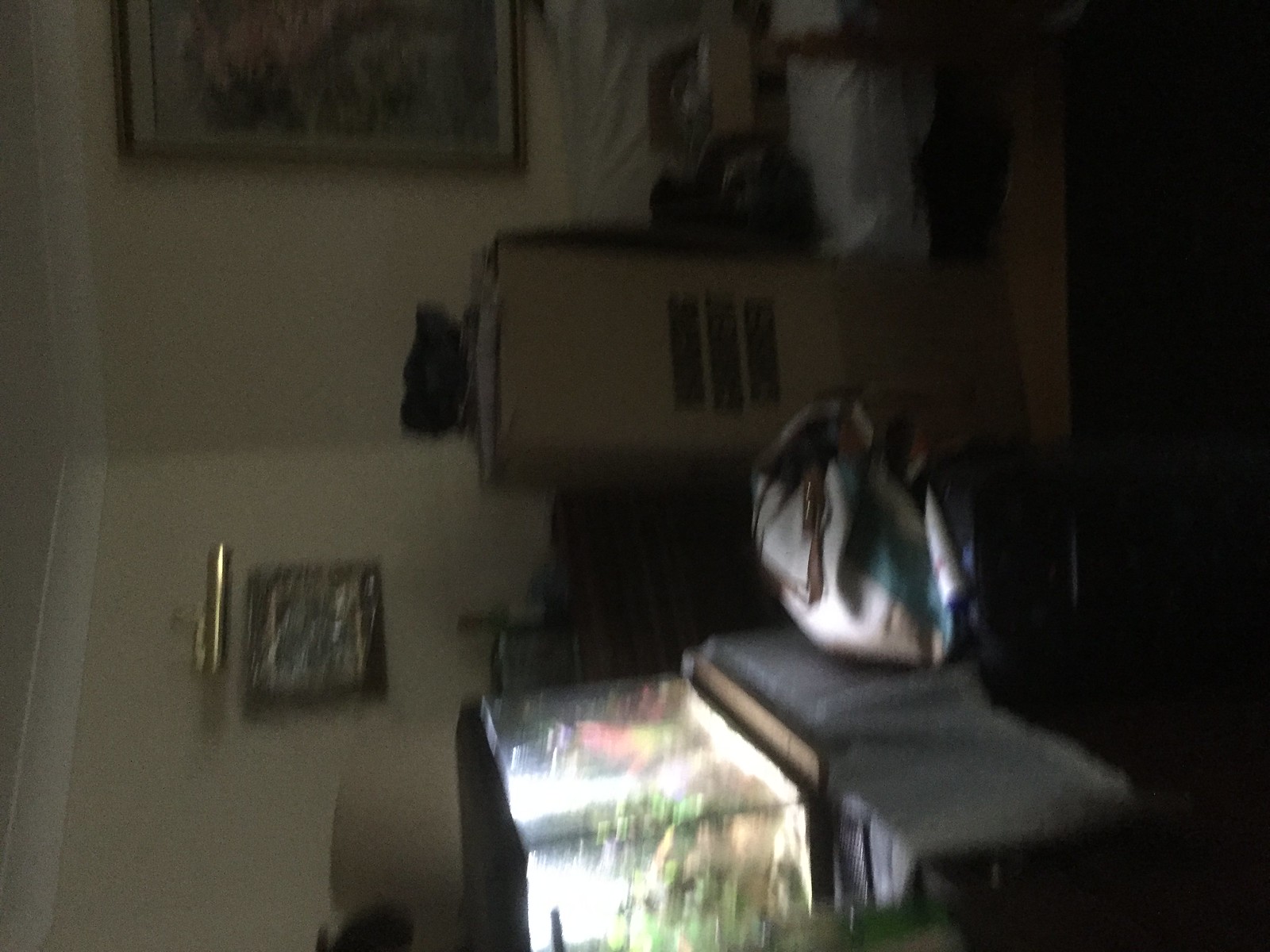A dim, blurry indoor photograph taken at an unusual angle, showing the corner of a room cluttered with various items. In the foreground, a brightly lit fish tank stands out, its rectangular shape and illumination contrasting sharply with the surrounding darkness. The right side of the image depicts the floor, while the left side shows the ceiling, emphasizing the photo's disorienting perspective. On the far wall, a framed painting hangs sideways, accompanied by an unlit light fixture above it. Scattered on the floor are a bag and some boxes, adding to the room's chaotic appearance. Another partially visible painting is also seen on the far wall, contributing to the eclectic mix of objects within the space.